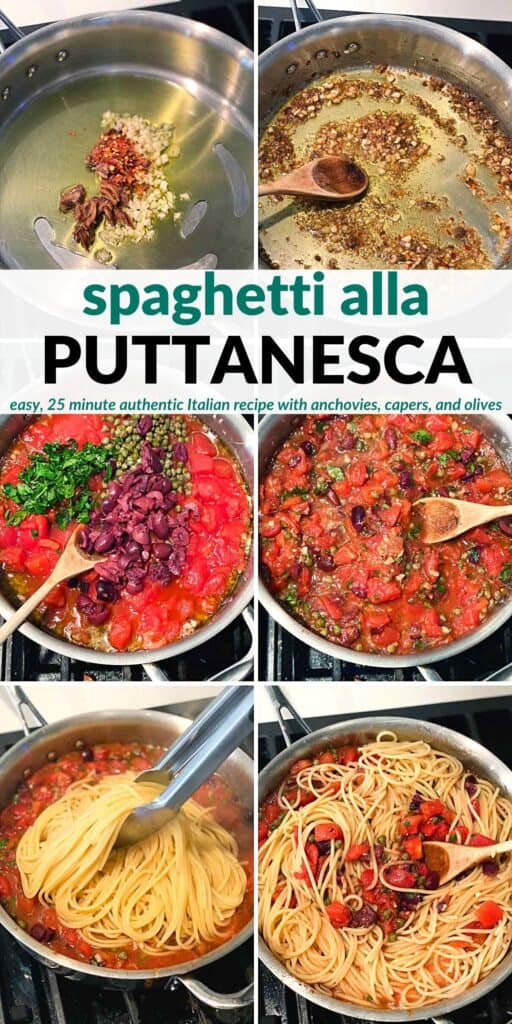The image is a detailed, step-by-step visual guide to making spaghetti alla puttanesca, an authentic Italian recipe that takes just 25 minutes. The center of the image prominently features the text in blue and black letters: "Spaghetti Alla Puttanesca," followed by "Easy 25-minute authentic Italian recipe with anchovies, capers, and olives."

The image is divided into six photographs, each illustrating a specific stage in the cooking process:

1. The first photo shows a stainless steel pan with olive oil, garlic, and various spices beginning to sizzle.
2. The second photo continues with the mixing of these ingredients, enhancing their aromatic qualities.
3. In the third photo, tomatoes, capers, olives, and potentially red onions and parsley are added to the pan, ready to be cooked together.
4. The fourth photo captures the sauce as it cooks and blends, with a wooden spoon stirring the ingredients to perfect the mixture.
5. The fifth photo shows the addition of cooked white spaghetti noodles directly into the rich, simmering sauce.
6. The final photo depicts the completed dish, with the pasta thoroughly mixed into the sauce, making a vibrant and delectable spaghetti alla puttanesca.

This descriptive guide provides a comprehensive visual and textual walkthrough, detailing the transformation from simple ingredients to a classic Italian dish.